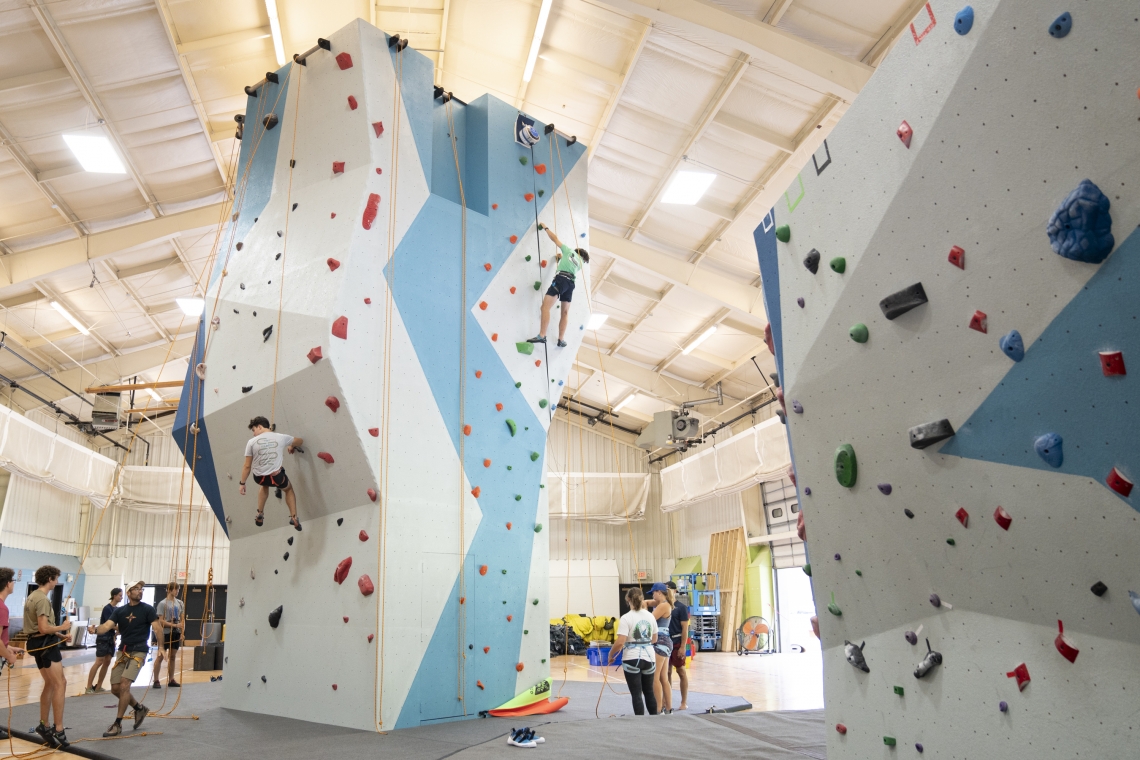The photograph captures the bustling interior of a brightly lit rock climbing gym, teeming with climbers and onlookers. Dominating the scene are large, man-made climbing structures with surfaces presenting a mix of irregular polygonal shapes and flat vertical walls, each decked with an array of multicolored climbing holds in various shapes and sizes, from footholds to handholds in hues of red, orange, green, and blue. The center stage is occupied by a towering climbing wall resembling a pretend mountain where two climbers ascend, each securely attached to ropes via harnesses for safety. The climber on the left seems to be descending, while the one on the right is still scaling the wall. Below, on protective mats covering the wood flooring, attentive belayers manage the safety ropes, ensuring the climbers' security. The high-ceilinged space, painted predominantly white with blue accents and featuring visible ventilation systems, houses other climbers waiting their turn and spectators observing the action, encapsulating a vibrant atmosphere of fun and fitness.